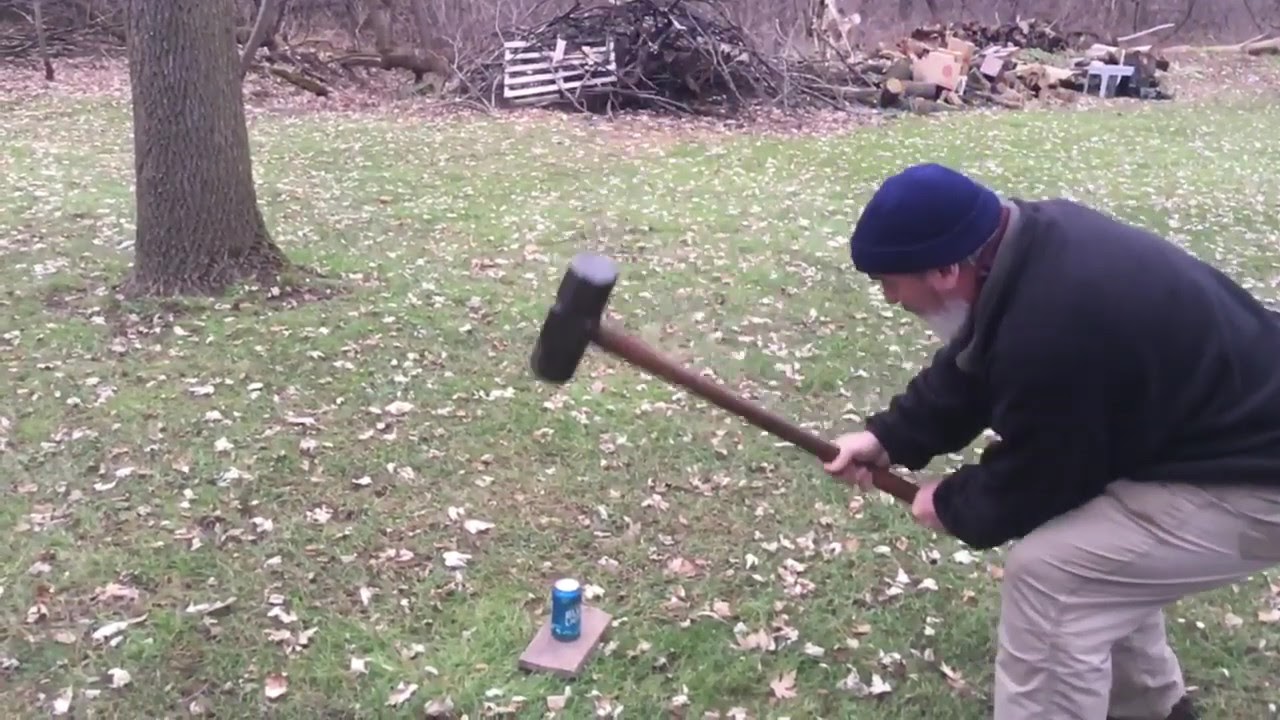In this picture, a man is standing on a grassy lawn covered with autumn leaves, holding a large sledgehammer. He has a navy blue beanie, a black sweatshirt, and tan khaki pants. Positioned on the right side of the foreground, he faces left, preparing to swing the sledgehammer towards an aluminum soda can—possibly Sprite—placed on a small board approximately 8 inches long and 6 inches wide. The sledgehammer's handle is brown, and the ends are black. The scene includes a slightly wooded area; to the top left, there’s a prominent tree trunk next to a piled heap of scrap wood, logs, a pallet, and other debris. The background extends to more trees without leaves, emphasizing the autumn setting.